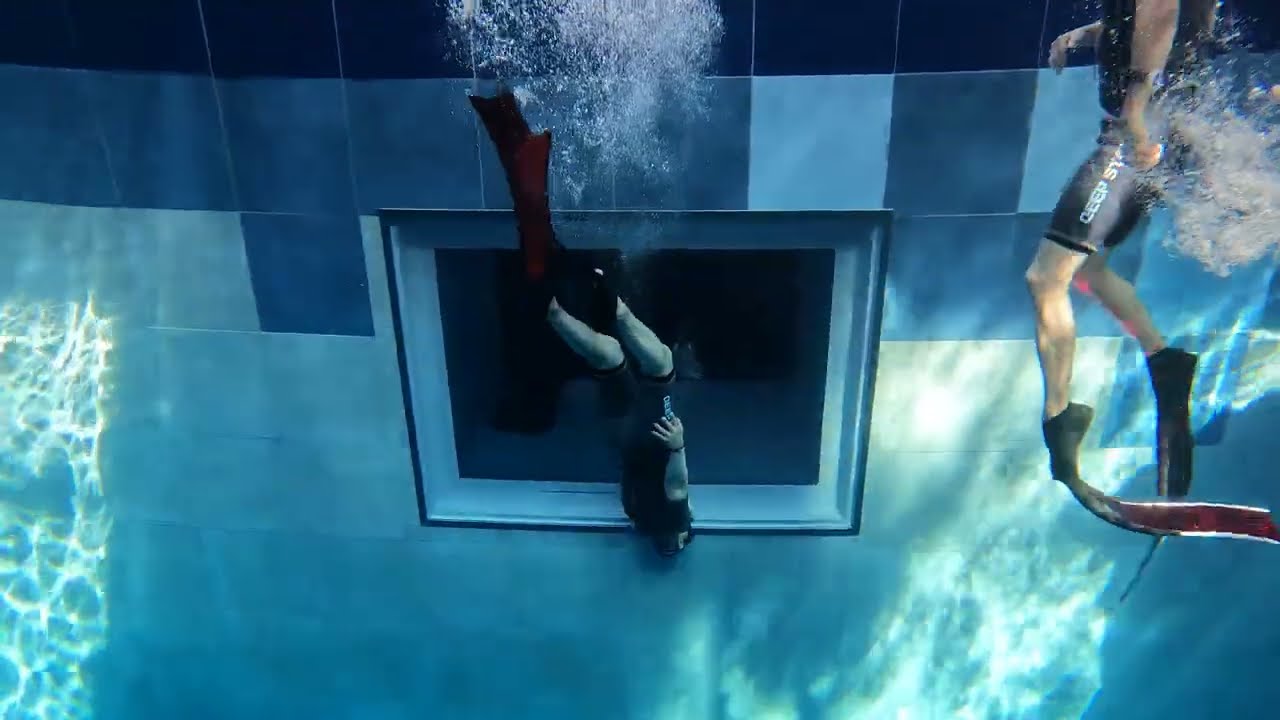This high-definition photograph, taken by an underwater camera, captures an intricate scene of two swimmers in a pool, possibly during a diving practice. The image is horizontally rectangular and showcases a swimmer on the left side, visible from the shoulders down, wearing tight-fitting bathing trunks adorned with blue and light yellow text that might read "DEEP." This swimmer is equipped with an air tank on their back and long fins on their feet. In the center of the image, another swimmer appears upside down, with their feet at the top and head at the bottom, also wearing long fins but lacking an air tank. The background reveals a pool wall composed of square tiles in varying shades of blue and white, with a prominent window suggesting an aquarium-like viewing area behind it. The colors predominantly include different shades of blue and white, enhancing the underwater ambiance.